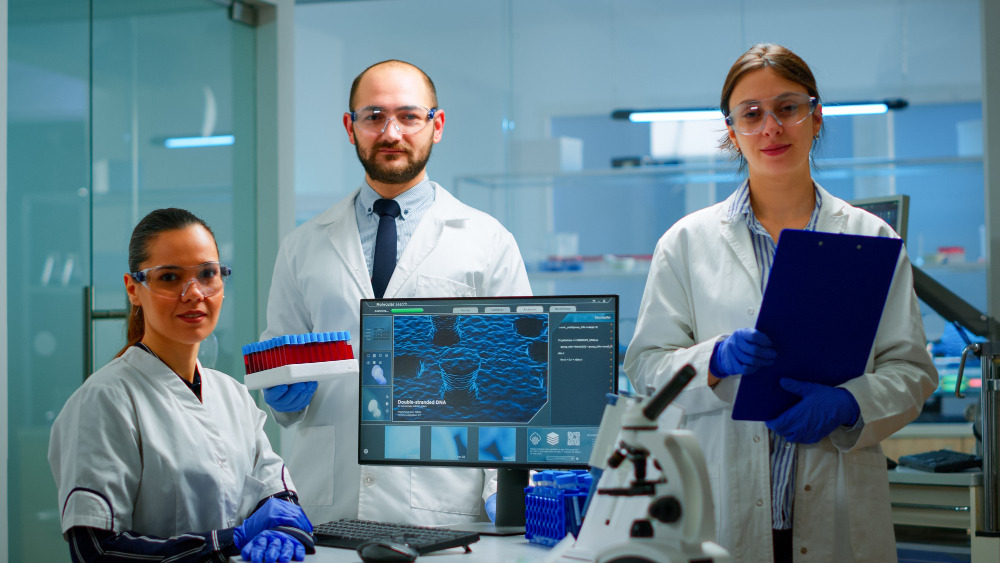The image captures a highly sterile hospital or laboratory setting with three individuals who appear to be scientists or doctors posing for the camera. Each person is equipped with safety goggles and blue latex gloves, emphasizing the clinical environment. On the left, a woman sits confidently, dressed in short-sleeved scrubs over a long-sleeved shirt, her hair pulled back into a ponytail. She appears to be in her late 20s or early 30s. In the center stands a man with a partially balding head, a beard, and a mustache. He is dressed in a light blue button-down shirt, a navy blue tie, and a white laboratory coat. He holds a white tray filled with vials, likely containing red liquid, capped in blue and red, which rest on a styrofoam platform. On his right, another woman stands poised with her hair neatly pulled back. She wears a light blue and white striped button-up shirt under an unbuttoned lab coat and holds a dark blue clipboard in both hands. The background is lined with clear glass doors and walls, showcasing an array of laboratory equipment, a computer monitor displaying a zoomed-in microscopic blue image, and other technical furnishings, all contributing to the precise and methodical atmosphere of the room.